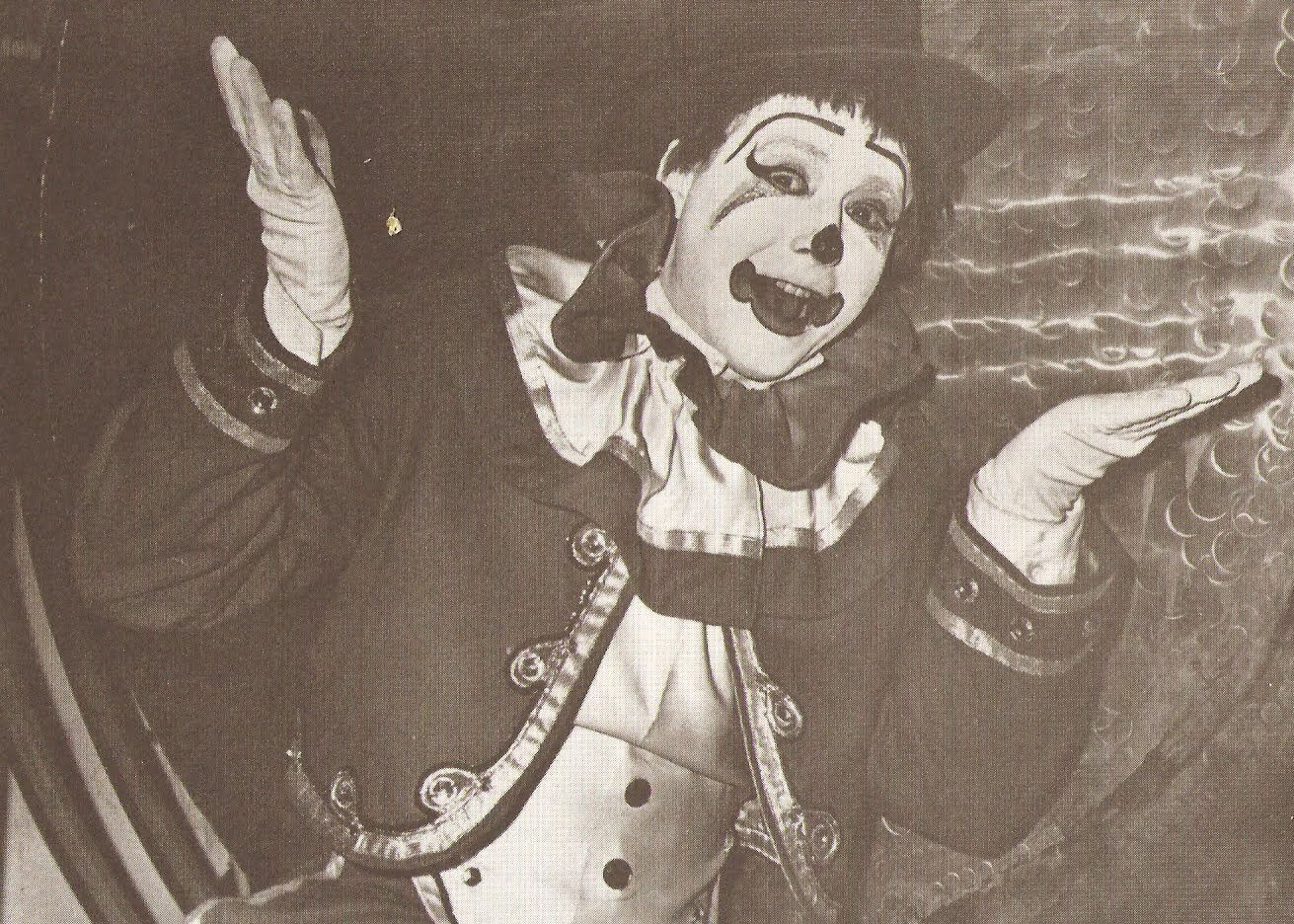This antique black-and-white photo, with a subtle sepia tone, captures an elaborately dressed clown standing before an indistinct, likely shiny, background that might feature a circus logo or metallic element. The clown's painted face, with a heavily outlined mouth showing a broad, toothy smile and darkened features including a bulbous nose and thick eyebrows, makes it hard to discern the person's gender. Dressed in a top hat and a fancy suit jacket adorned with shiny buttons, the clown also wears a flowy, ruffled collar and white gloves. Posing with hands raised in a shrug-like gesture, as if saying "I don't know," the clown exudes an air of cheerful ambiguity. The overall look is completed by a buttoned vest and an impression of vintage circus flair, reminiscent of a figure straddling the roles of both a clown and a ringmaster.